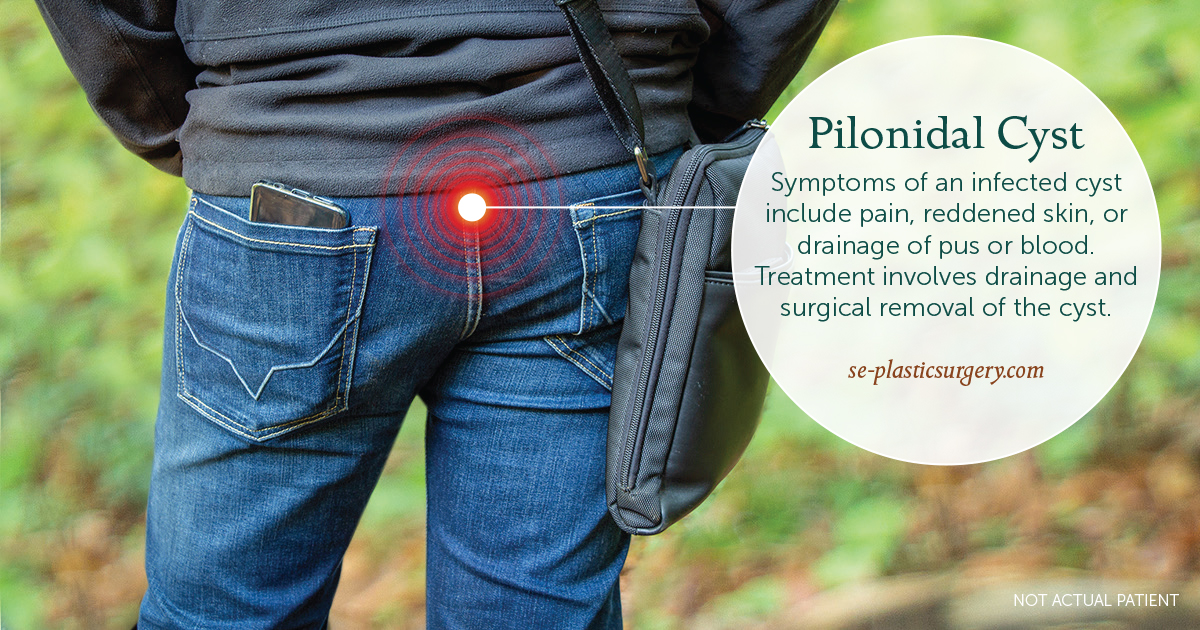The image is an informational advertisement about pilonidal cysts, prominently featuring a partial view of a man from the back. He is positioned against a blurry forest background with green vegetation, emphasizing his figure. He is dressed in a dark gray hoodie, blue jeans, and is carrying a dark gray messenger bag with brass rivets. A cell phone is partially visible in his left back pocket. The jeans display creases from his stance. Central to the image is a bright red dot located at the lower back, around the tailbone area, illustrating the typical location of a pilonidal cyst. The focal point is encapsulated within a circular white graphic, accompanied by an informational text that details symptoms—pain, reddened skin, and drainage of pus or blood. It also outlines that treatment involves drainage and surgical removal of the cyst. The text includes a URL, "se-plasticsurgery.com," and a note that reads, "not actual patient," to clarify the illustrative nature of the image.